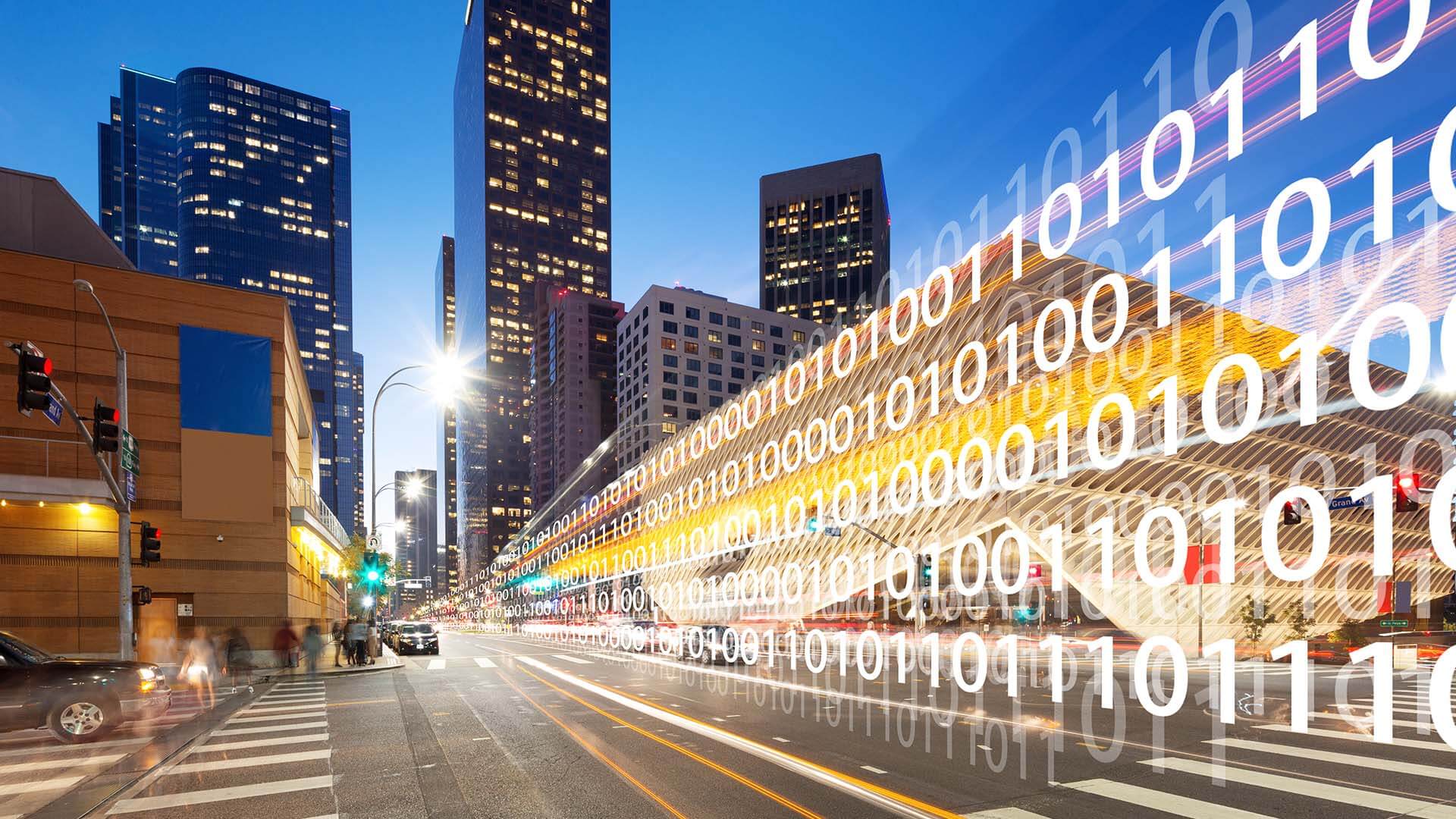A vibrant city street stretches into the distance under a clear, bright blue sky, resembling the graphical style of a video game. Dominating the skyline are three towering high-rise buildings illuminated by numerous yellow lights, with smaller structures nestled below them. In the foreground, a prominent brown building stands next to a bustling roadway.

The street is lined with vehicles, some seemingly parked or possibly stopped, hinting at a moment of pause in the city's perpetual motion. A green traffic light indicates the direction of traffic flow, while a car on the left waits at a red light. Pedestrians cross the street, navigating the clearly marked white crossing lines.

On the right side, a blur of white binary numbers – 011, 010, 1100, 101 – overlays the scene, running continuously down the street, contributing to the digital aesthetic of the image. This juxtaposition of urban life and digital elements captures the essence of a modern, possibly futuristic, metropolis.